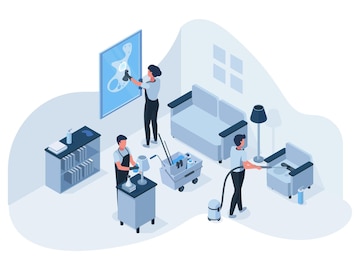This is a digitally generated image resembling a cartoon, depicting a meticulously detailed office space in shades of grayish blue. The scene focuses on a trio of cleaners actively tidying the room. The floor and walls share a light blue hue, creating a cohesive atmosphere. 

In the background, to the left, a woman with dark hair, dressed in a light blue shirt and black pants, is cleaning a blue painting adorned with light blue splotches. Her back is to the viewer. Below the painting, a light blue couch with black armrests is positioned, and above it, four petite windows allow a glimpse of the outside. 

Adjacent to the couch is a light blue chair with dark blue armrests. A man with short dark hair, also wearing a light blue shirt paired with blue pants, is vacuuming the chair. His stance is slightly side-on, revealing his earnest engagement with the task at hand. Nearby, a cart brimming with an array of cleaning supplies stands ready for use.

Towards the right, there is a light blue table with black legs and a blue top. On the table sits a lamp and a cup. A male cleaner, characterized by his short black hair and attire consisting of a light blue shirt and a black apron, is seen wiping down the lamp with a blue towel. 

To the left of the painting, a small black-topped shelf houses an assortment of books, including a noticeable white book. Scattered around the space are cleaning essentials including a mop bucket, bookcase, and vacuum cleaner, further emphasizing the ongoing activity of keeping the area spotless.